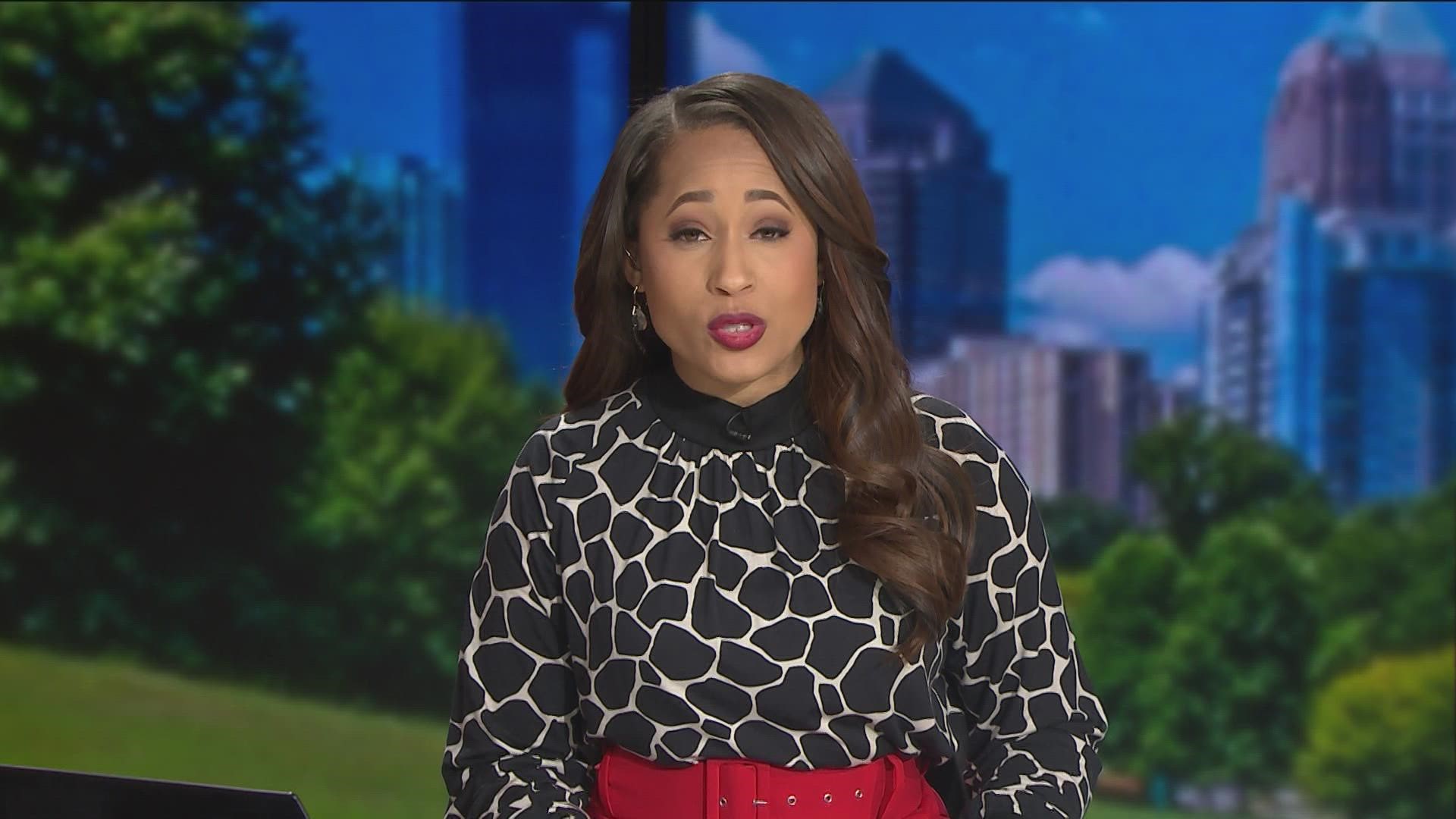In this image, we see a woman who appears to be a newscaster delivering a news story. She has a fairly tanned complexion, which suggests she might be of mixed Asian or African American descent. Her long brown hair and makeup, which includes lipstick and eye shadow, make her look camera-ready. She has a serious expression on her face, with her eyebrows lifted and a slight crease in her forehead, indicating she might be speaking mid-sentence.

She is wearing a black and white geometric patterned long-sleeve blouse with a black collar, paired with a striking red belt or possibly a red skirt. The image captures her from the waist up, focusing on her and slightly blurring the background.

The background appears to be a cityscape with towering high-rise buildings on one side and lush green trees and grassy areas on the other, suggesting a park. It is uncertain whether the background is real or a projected image on a green screen, but it enhances the sense of a metropolitan setting. The woman's position directly facing the camera and her attire strongly emphasize her role as a professional newscaster.